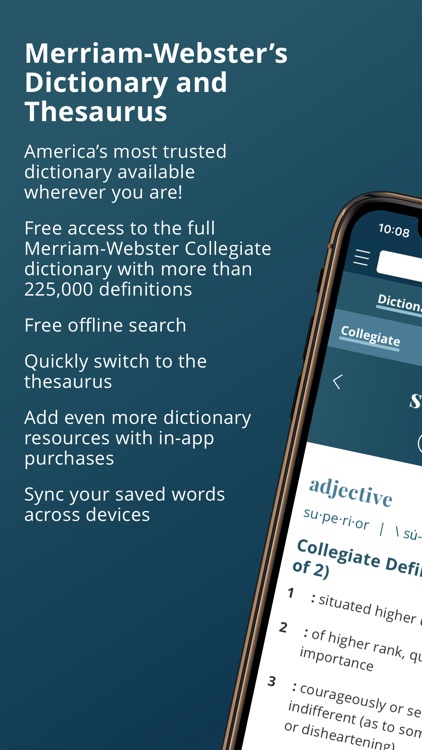This photo is likely an advertisement for Merriam-Webster's Dictionary and Thesaurus. The text prominently states "America's Most Trusted Dictionary available wherever you are," highlighting features such as free access to the full Merriam-Webster Collegiate Dictionary, which boasts over 225,000 definitions. Additional attributes include free offline search, quick Thesaurus switching, in-app purchases for additional resources, and the ability to sync saved words across devices. On the right side of the image, a smartphone is visible, displaying a portion of the dictionary interface with the time shown as 10:08 AM. The screen shows part of a definition, reinforcing the accessibility and comprehensive nature of the digital dictionary.